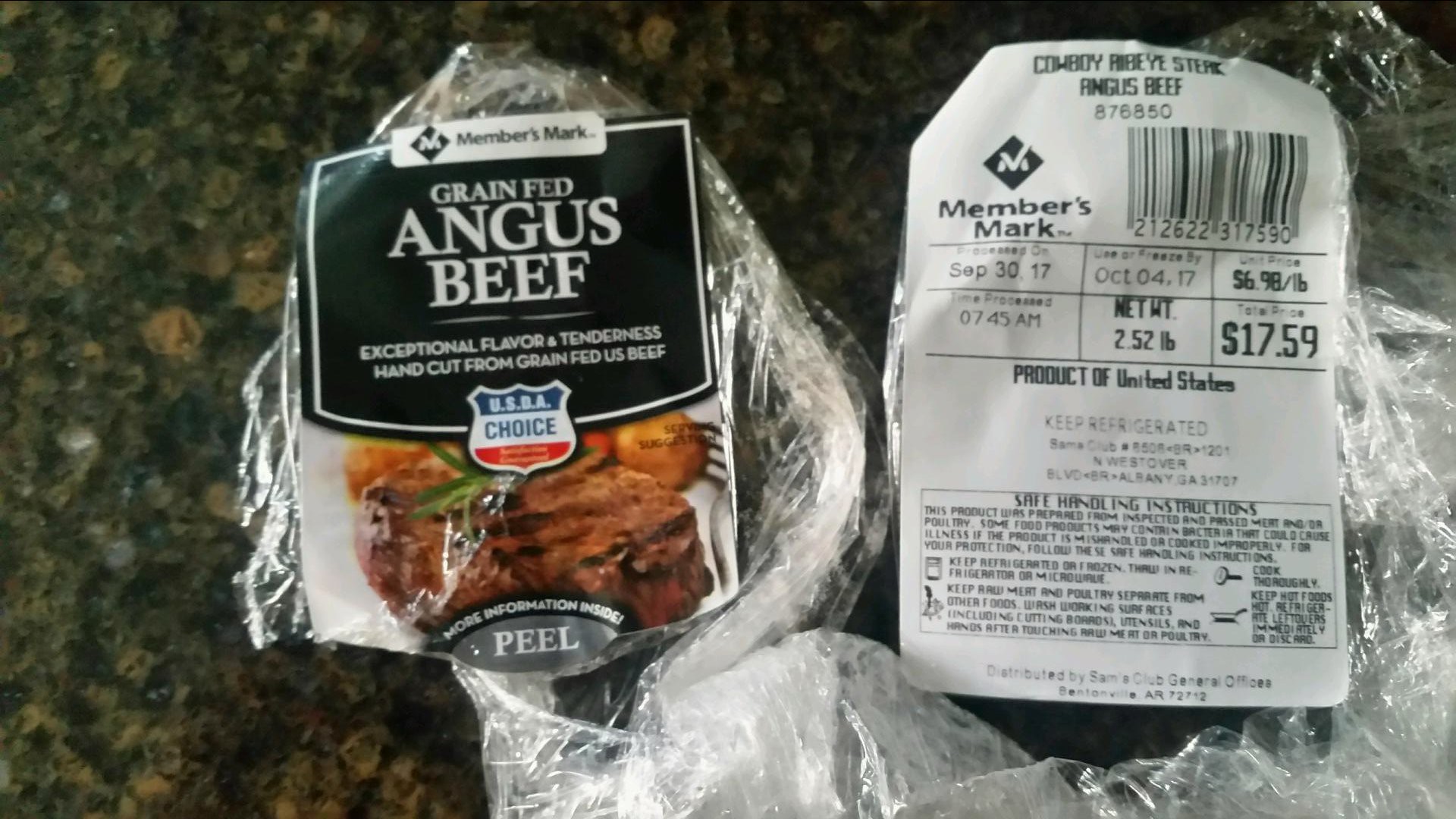This image prominently features the packaging for a purchase of grain-fed Angus Beef, showcased with the Member's Mark sales logo. The packaging flaunts a reputation for exceptional flavor and tenderness, highlighted by hand-cut, USDA Choice U.S. beef. A distinct label invites consumers to peel for additional information.

On the right side of the packaging, specific product details are printed: it's identified as Cowboy Ribeye Steak, catalog number 876850, and packed on September 30th at 7:45 a.m. Consumers are instructed to use or freeze the beef by October 4th. We see it weighs 2.52 pounds, priced at $6.98 per pound, totaling $17.59 for this purchase. The packaging states it's a product of the United States and emphasizes the importance of keeping the beef refrigerated, accompanied by safe handling instructions.

The scene where this packaging lies suggests a home kitchen environment, as indicated by the marbleized stone-like countertop, typical of a food preparation area. While the plastic wrapper and labels are visible from both the front and back, the actual beef remains concealed within the packaging.